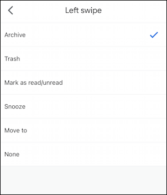The image is a minimalist screenshot captured in portrait mode, featuring a predominantly white background with a subtle gray gradient near the bottom. The entire screenshot is bordered by a very light black outline. 

In the upper left-hand corner, there is a back arrow icon. Centered at the top, the text reads "Left Swipe." Below this, the first row displays the word "Archive" with a blue check mark to its right, indicating that the "Archive" option is currently selected. 

The subsequent rows list other options without any selections. These include:
- "Trash" in the second row
- "Mark as Read/Unread" in the third row
- "Snooze" in the fourth row
- "Move to" in the fifth row
- "None" in the sixth row

The image appears to be a UI screenshot from an application, likely demonstrating user settings for what action will be performed when an item is left-swiped. In this instance, left-swiping an item will result in it being archived.